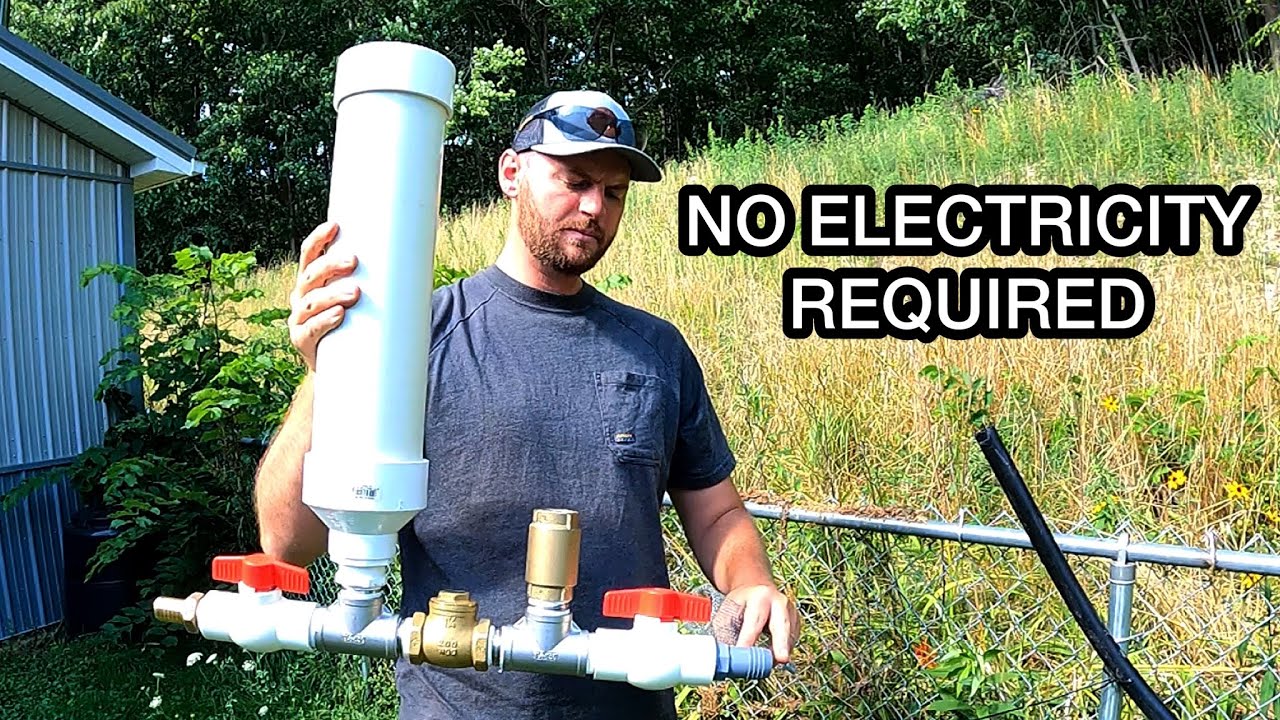In the image, taken outdoors during the daytime, a man stands central, looking down at something in his hand. He is a white male, approximately 35 to 40 years old, dressed in a grey cotton t-shirt and a grey baseball cap with sunglasses draped over the front. The man sports a short, scruffy brown beard. He appears to be a contractor or plumber, showcasing a PVC pipe system connected to metal pipes—both silver and gold—featuring several valves and orange levers that suggest a pressure valve system. Behind him, a silver chain link fence about three feet tall separates him from the background, which includes a lot of dark green trees, tall overgrown grass, weeds, and a shed on the left side of the image. There’s visible text on the right side of the photo that reads "no electricity required" in white letters with a black outline.